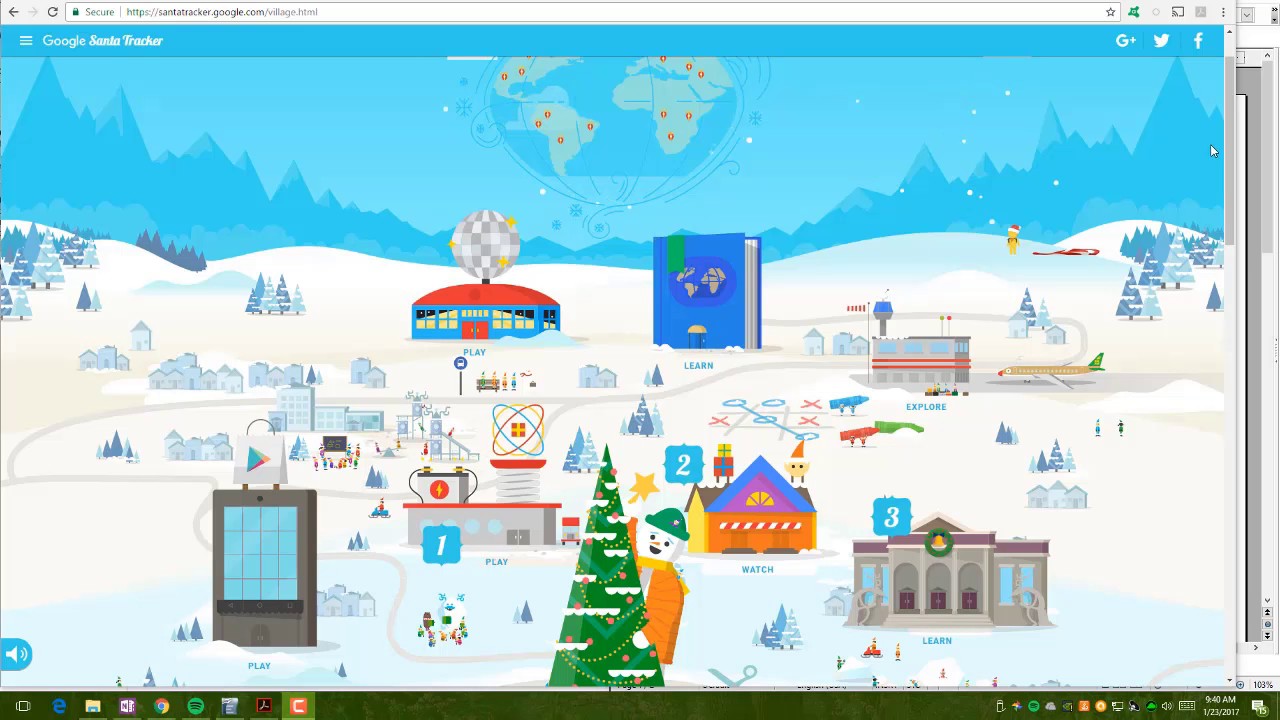The screenshot depicts a winter-themed user interface, dominated by a light blue banner stretching across the top. This banner reads "Google Santa Tracker" and is flanked by three social media icons on its right side: the old Twitter bird logo, the Facebook logo, and the Google Plus (G+) logo. Although there's a URL at the very top, its text is too small to discern.

Below this banner, the web page presents a whimsical cityscape adorned for the holiday season. Central to the scene is a small Christmas tree surrounded by a snowman, adding a festive touch to the middle ground. On the right side of the background, there's a towering book, while the left side features a building topped with a large disco ball, adding a quirky element to the winter scenery. Above this enchanting city scene, a globe floats in the sky, contributing to the magical atmosphere of the webpage.